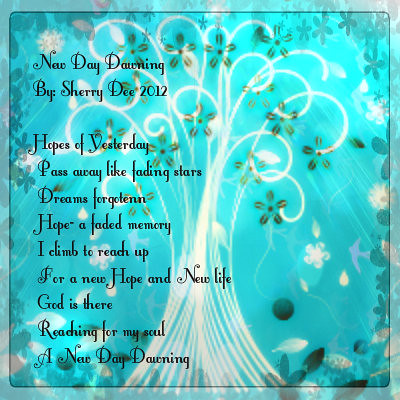This image features a square graphic that closely resembles a piece of digital artwork. The background is an enchanting turquoise-blue, with whimsical, curling white lines forming an ethereal tree-like illustration. Tiny star-shaped flowers and green leafy details accentuate the tips of the white branches, adding to the dreamy aesthetic.

Central to this design is a poignant, cursive black text, neatly positioned on the left side. The text reads: "New Day Dawning" by Sherry D., dated 2012. The short poem featured on this artwork conveys a sense of renewal and spiritual optimism. It reads: "Hopes of yesterday pass away like fading stars, dreams forgotten, hope a faded memory. I climb to reach up for a new hope and a new life. God is there reaching for my soul, a new day dawning." The overall feel of the image is serene and reflective, possibly intended for sharing on social media or as the front of a sentiment-laden card.